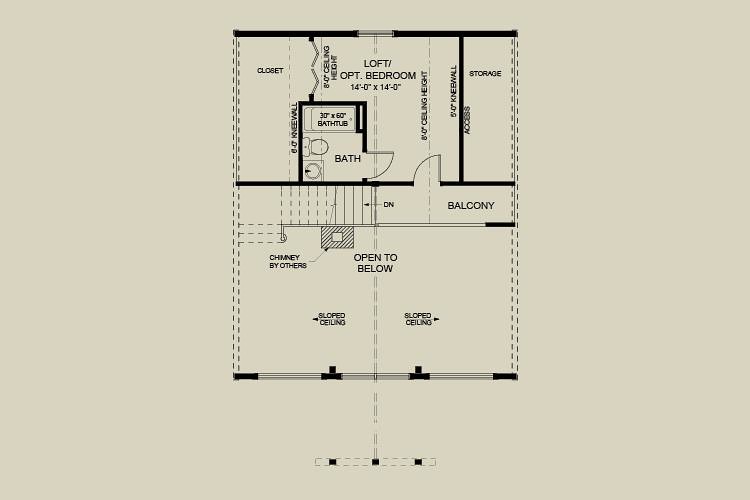The image depicts a detailed floor plan on manila-colored paper, displaying a loft/optional bedroom. The plan showcases a rectangular layout with a black wall at the top and a central doorway, likely the front entrance. The loft/optional bedroom area is labeled with dimensions 14'-0" x 14'-0". Adjacent to this space on the left is a squiggly feature and a closet. Below the loft area, there's a black square marked "bath", illustrating a bathroom equipped with a toilet, sink, and a 30" x 60" bathtub.

To the right of this bath area is a storage space within a black rectangular section, complete with a door leading to a balcony. Stairs descend from this point, accompanied by a note indicating "chimney by others", leading to an "open to below" space. The plan designates sloped ceilings on both halves of this lower area. Outside the rectangular confines, a dashed-line rectangle with black squares is also present.